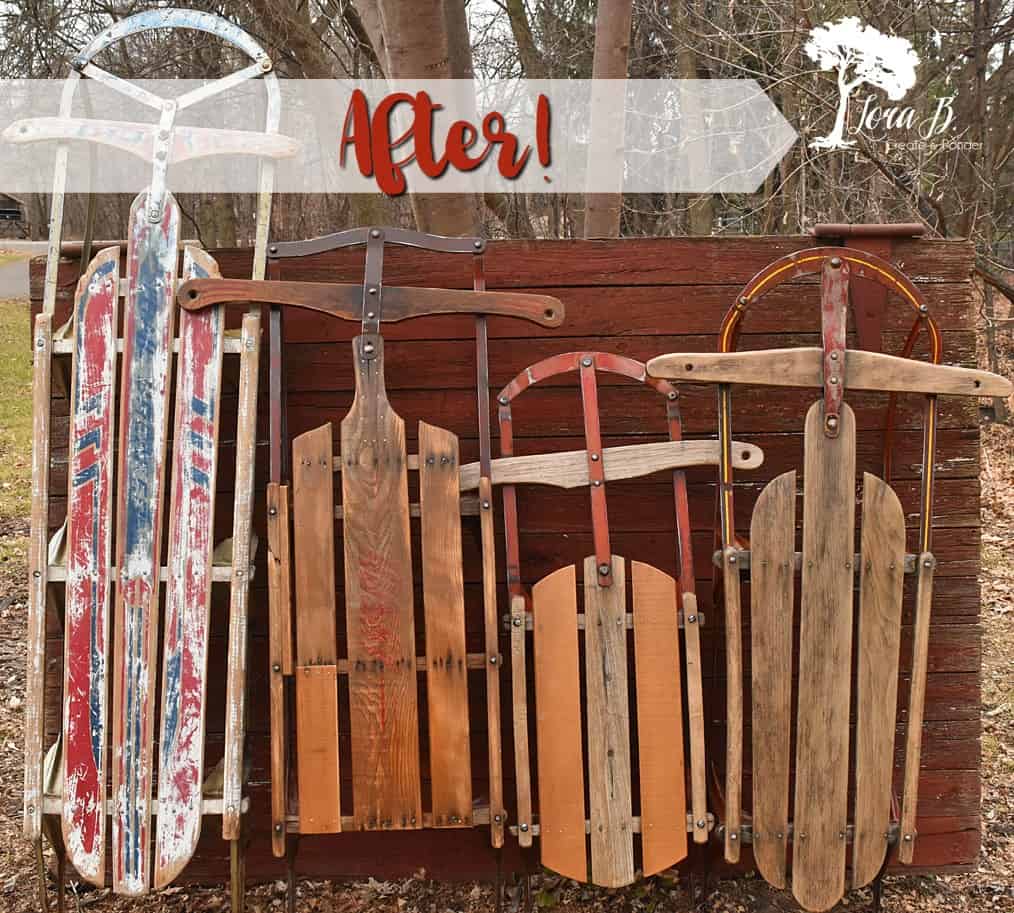This photograph captures a nostalgic outdoor scene featuring four old sleds displayed leaning vertically against a wooden fence in an open field. The sled on the far left is the tallest and once showcased vibrant red, white, and blue colors, now worn and faded with age. The next three sleds to the right are progressively shorter, made of wood, and exhibit signs of rusted metal and wear. The smallest sled in the center, although newer-looking than the others, still has an aged appearance. Each sled is a different style, adding to the eclectic historic display. In the background, bare trees indicate an off-season with no snow in sight. At the top of the image, there is peculiar red text with an exclamation point atop a white arrow, pointing toward a tree marked with the name "Laura B." The weathered look of the sleds and the muted tones of the surrounding environment evoke a sense of nostalgia and the passage of time.